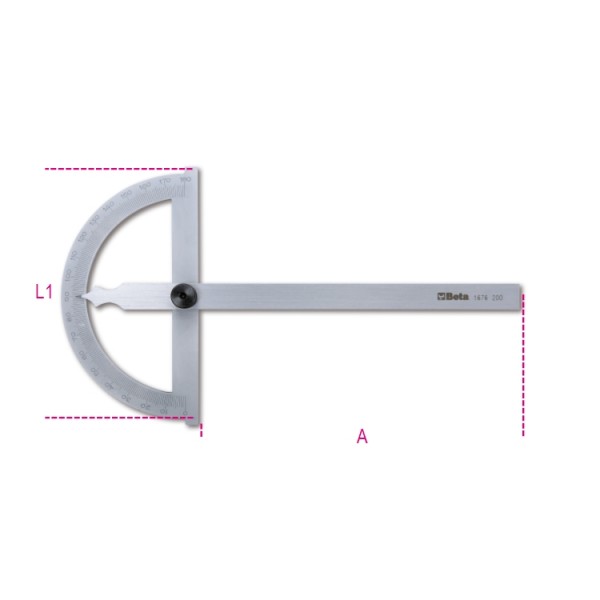The image depicts a detailed diagram of a protractor-based measuring instrument, positioned vertically with its curved half-moon shape oriented to the left and all markings facing outward. The vertical flat part of the protractor has a plain, metallic appearance. Attached centrally to the protractor by a black circle is a long, flat metal rod. This rod extends horizontally and possesses a pointed, indented edge nearing the protractor's curved part on the left side. The diagram is annotated with labels in a reddish-purple color: "L1" is marked at the crest of the protractor's curve, and the letter "A" is situated at the bottom right, beneath the rod. Three reddish-purple dashed lines run horizontally at the top and bottom and vertically along the right edge of the rod, contributing to the instrument's measurements. The rod features the text "beta," next to which appears the sequence "1676" and "200." There is also a logo near "beta," possibly resembling two leaves.